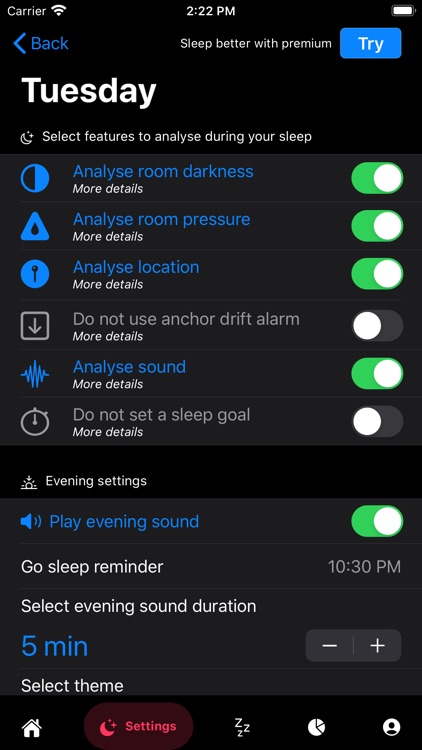This is a highly detailed screenshot from a cell phone screen displaying a sleep tracking app interface. The background is entirely black. 

At the top:
- In the top left corner, it reads "Carrier" in white.
- Next to it, the WiFi icon shows full bars, also in white.
- Centered at the top, the time "2:22 PM" in white text.
- On the top right, there’s a battery icon.

Beneath the "Carrier":
- A blue arrow pointing left accompanies the word "Back" in blue text.

Centered under the time:
- The text "Sleep Better with Premium" in white.

To the left of the battery icon:
- A blue tab with the word "Try" in white.

Below the "Back" button:
- Bold white text reading "Tuesdays."
- Next to a small nighttime icon, there is text in white: "Select features to analyze during your sleep."

Further down:
- A gray square on the left contains six blue and black icons:
  1. A semi-circle split into gray and dark blue.
  
To the right of these icons:
- Each icon has blue text with smaller white text beneath it.
- On the right side, green-background toggles (with white sliders) control various features:
  - The top three toggles are turned on.
  - The fourth toggle is turned off.
  - The fifth toggle is on.
  - The sixth toggle is off.

A black-bordered section:
- Includes the text "Evening settings," next to a sunrise icon.

Below this section:
- Another small square features a sound icon and blue text "Play evening sound," which is toggled on to the right.

Further details:
- White text "Go sleep reminder" and the time "10:30 PM" on the right.
- The option "Select event duration" with blue text "5 min" beside a white minus and plus sign in a rectangle.
- Text "Select theme" below this.

At the bottom:
- An inch of black border which contains:
  - A white home icon.
  - Red settings icon with a half moon.
  - Three white "zzz".
  - A white circle.
  - A white account icon.

This detailed description captures the complexity of the app interface and the various available features and settings.